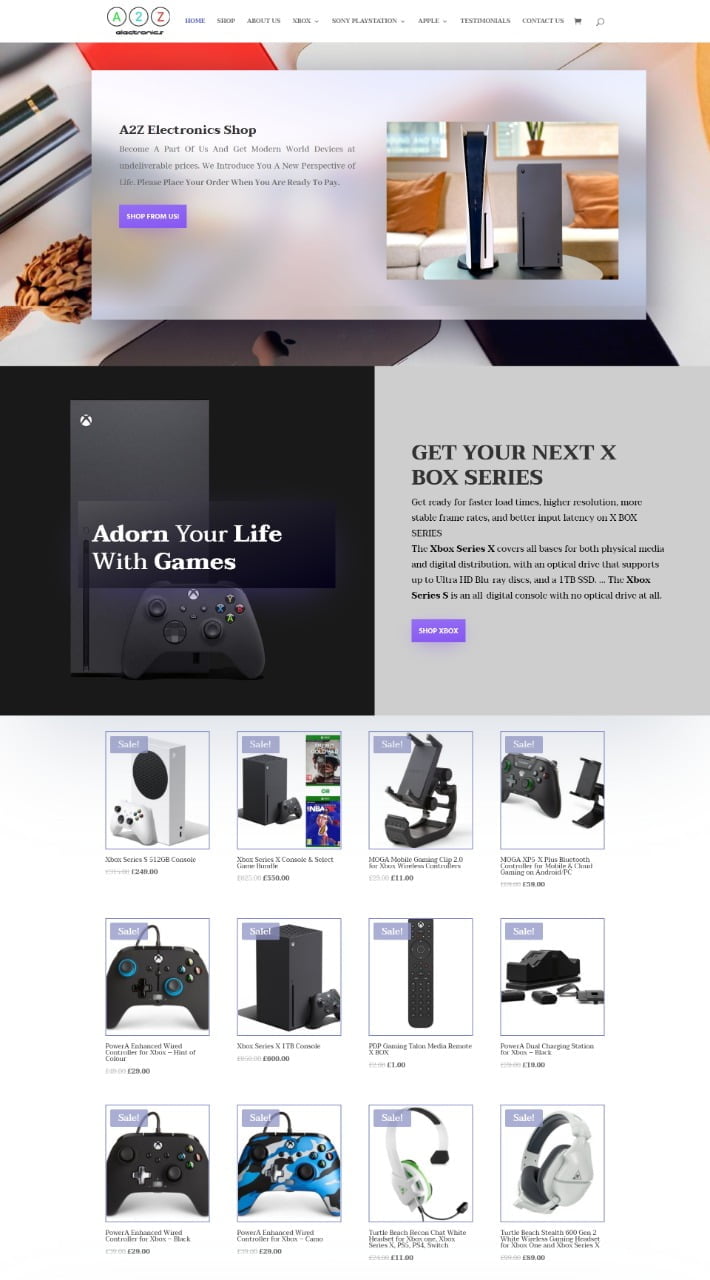This is a detailed caption for the screenshot from a website:

The top section of the screenshot features three circular icons: a green "A," a blue "2," and a red "Z." Adjacent to these icons is a navigation menu comprised of several tabs. The first tab is blue and labeled "House." Following tabs are in black text and labeled as "Shop," "About Us," "Xbox" (with a gray drop-down arrow), "Sony PlayStation" (with a gray drop-down arrow), and "Apple" (with a gray drop-down arrow). Additional navigation includes "Testimonials," "Contact Us," a shopping cart icon in black, and a black magnifying glass icon.

Below the navigation menu is a light gray section displaying circular mascara-type pens, one of which is highlighted with a gold banner. A red trapezoidal shape is also present in this area. A pop-up window in alternating bands of light and dark gray showcases a PlayStation 5 beside an Xbox One X. The PlayStation 5 has a black center with white sides, while the Xbox One X is dark gray all around. These gaming consoles are placed on a round black table next to a cream-colored couch against an off-white wall with windows and plants. The couch is adorned with orange pillows.

The central banner of the webpage features bold black text that reads "A2Z Electronics Shop." Below this, regular black text states, "Become a Part of Us and Get Modern World Devices at Undeliverable Prices. We introduce you to a new perspective of life. Please place your order when you are ready to pay." A rectangular purple button with bold white text says "Shop From Us."

The lower portion of the screenshot highlights an Xbox One X with a black controller in front of it, accompanied by large bold white text: "Adore in Your Life with Games." The words "Adore" and "Games" are in bolder white text than "Your" and "With." Additional bold black text reads "Get Your Next Xbox Series," followed by regular black text that advertises the console's features: "Get Ready for Faster Load Times, Higher Resolution, More Stable Frame Rates, and Better Input Latency on Xbox Series."

The subsection continues with bold black text introducing the "Xbox Series X," noting, "covers all bases for both physical media and digital distribution with an optical drive that supports up to Ultra HD Blu-ray Disc and 1TB SSD…" It also mentions the "Xbox Series S" in bold black text, describing it as "an all-digital console with no optical drive at all." The various systems and their respective price points are displayed at the bottom of the page.